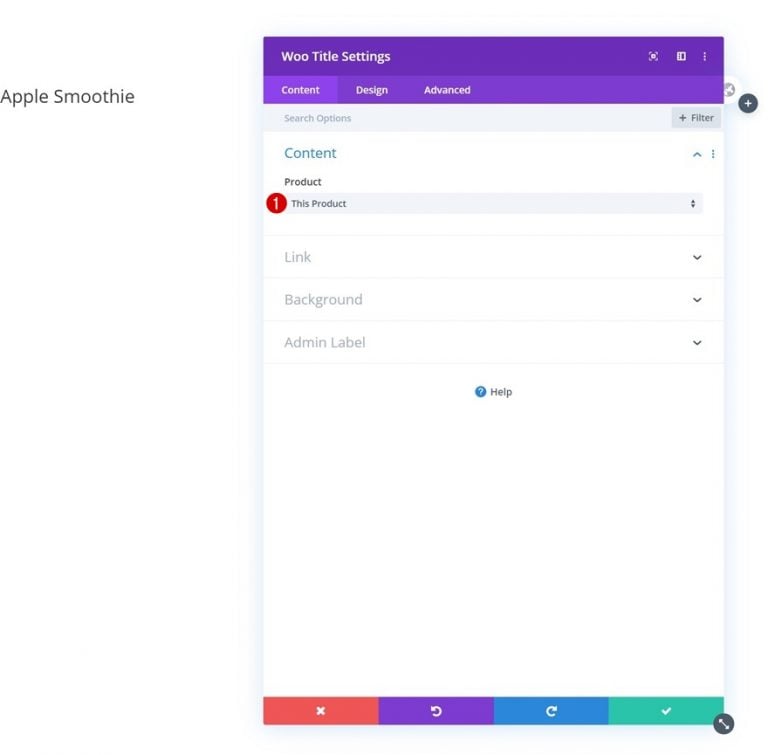The image showcases a user interface with distinct sections and controls. At the top, there's a dark purple border labeled "Woo Title Settings," featuring an X icon on the right for closing, a maximize icon, and an ellipsis for more options. Below this, a lighter purple area presents three clickable tabs titled "Content," "Design," and "Advanced."

On the left side of the interface, the text "Apple Smoothie" is displayed. Beneath the purple sections, there is a gray bar labeled "Search Options" with a "Filters" button to its right.

In the central part of the image, a white box prominently displays the word "Content" in blue lettering at the top. Below this, the word "Product" is shown, followed by "This Product" inside a gray box. Accompanying this is a red circle with the number one in the center, indicating a notification or item count.

Further down, the interface includes a "Link" label with an associated drop-down menu, followed by a "Background" label, also with a drop-down menu. Lastly, there is an "Admin Label" section with an additional drop-down menu and a "Help" button located at the bottom of the interface.